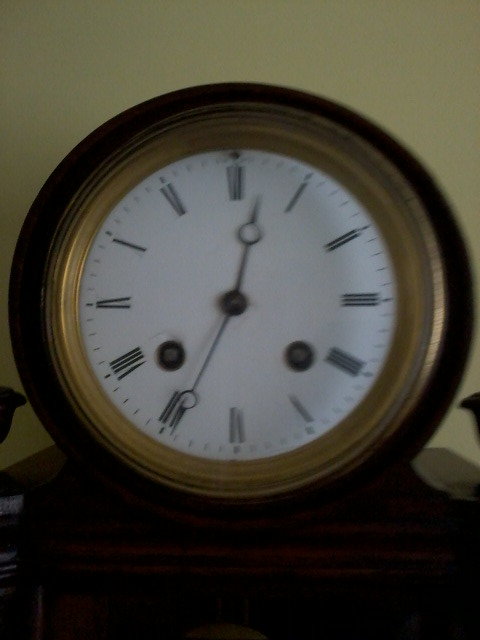In this image, a clock with a bronze or brown border is prominently displayed atop a brown pedestal, likely part of a bookcase. The clock's face is white, featuring black Roman numerals and black hands. Notably, there are two button-like dots near the 8 o'clock and 4 o'clock positions, whose purpose is unclear. The backdrop is a wall that appears to be either beige or white, but discerning the exact color is challenging due to the dim lighting that envelops the room.